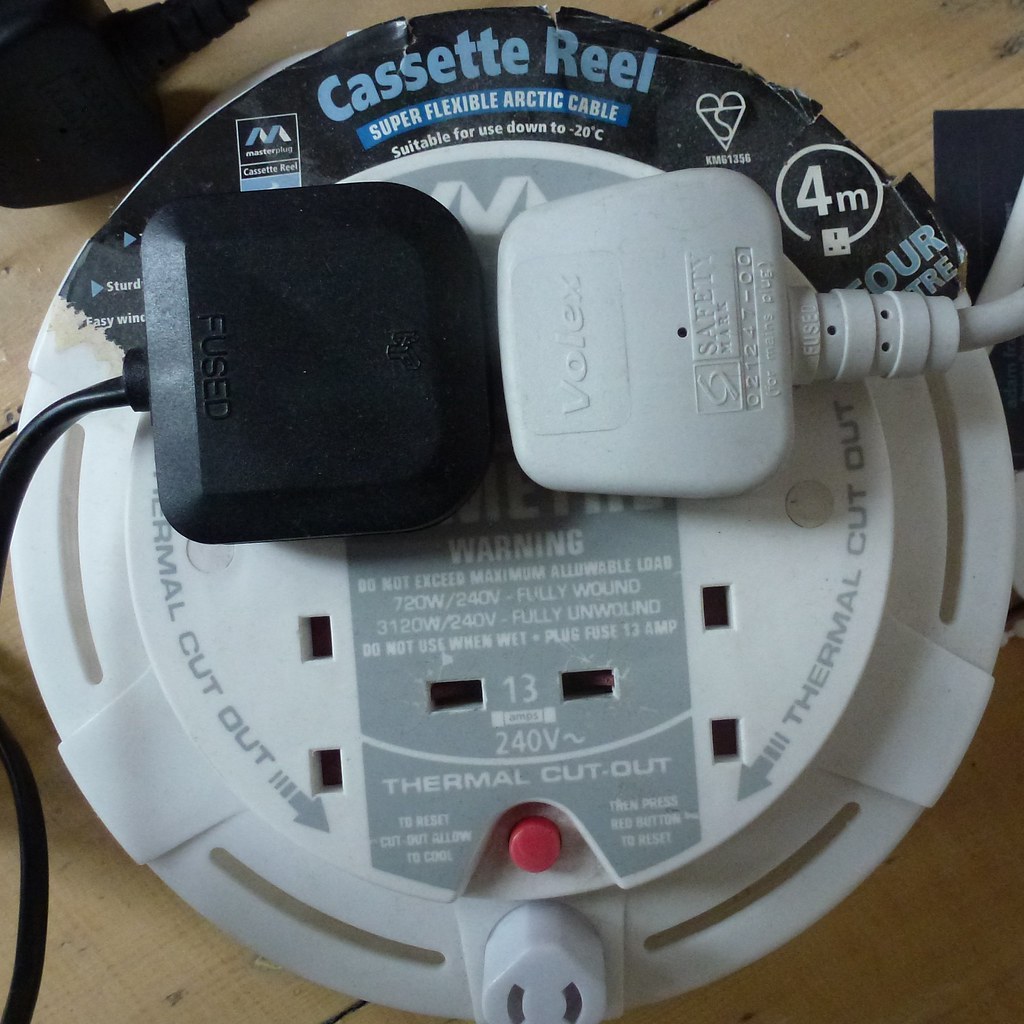This detailed image depicts an indoor scene of a circular extension cord placed on a light brown wooden surface. The extension cord, made of off-white plastic, features a central blue-green stripe with the text "Warning, do not exceed maximum allowable load." Above this, the label reads "Cassette Reel, Super Flexible, Arctic Cable, suitable for use down to -20°C." At the very top of the device is a black banner displaying company logos.

Two devices are plugged into the top outlets: a black, square-shaped plug marked with "Fused" and a white, trapezoidal plug labeled "Volex." Each plug has a wire extending out, with the black plug's wire curling to the bottom left corner and the white plug's wire extending out to the right. The base of the extension cord features a small red button near the bottom center, with "Thermal Cutout" printed above it, indicating a safety feature of the device. There are a total of four available outlets on the circular base, with two currently in use and two remaining free.